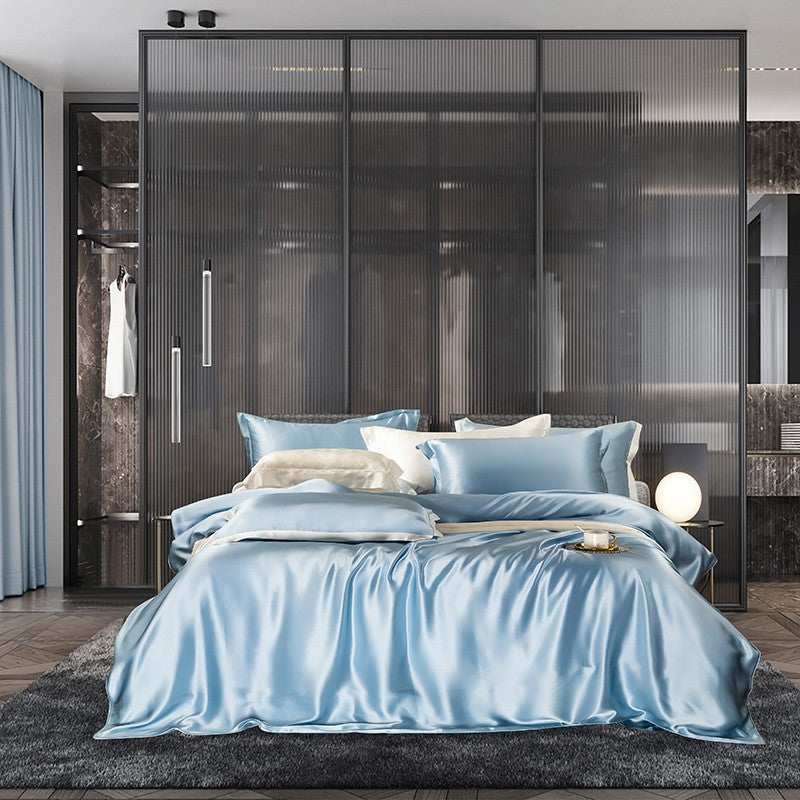The photograph showcases an upscale, modern bedroom with a luxurious design. The main focus of the image is the bed, which is elegantly made with baby blue silky sheets and sky blue and white pillows generously arranged at the head. The bed is set on a plush, dark gray rug that rests atop a beige tile floor, with just a hint of wooden flooring visible at the rug's borders. To the right side of the bed, a low nightstand holds an illuminated globe lamp, adding a warm touch to the contemporary setup. A tray with a coffee cup and spoon is positioned at the foot of the bed. Behind the bed, three panels of frosted glass, framed in black metal with vertical lines, partially obscure a closet filled with black and white clothing and a giant mirror equipped with a light. The left edge of the image hints at floor-to-ceiling light blue curtains that complement the bedspread. The overall aesthetic of the room is very modern and luxurious, with attention to detail that highlights its sophisticated design.